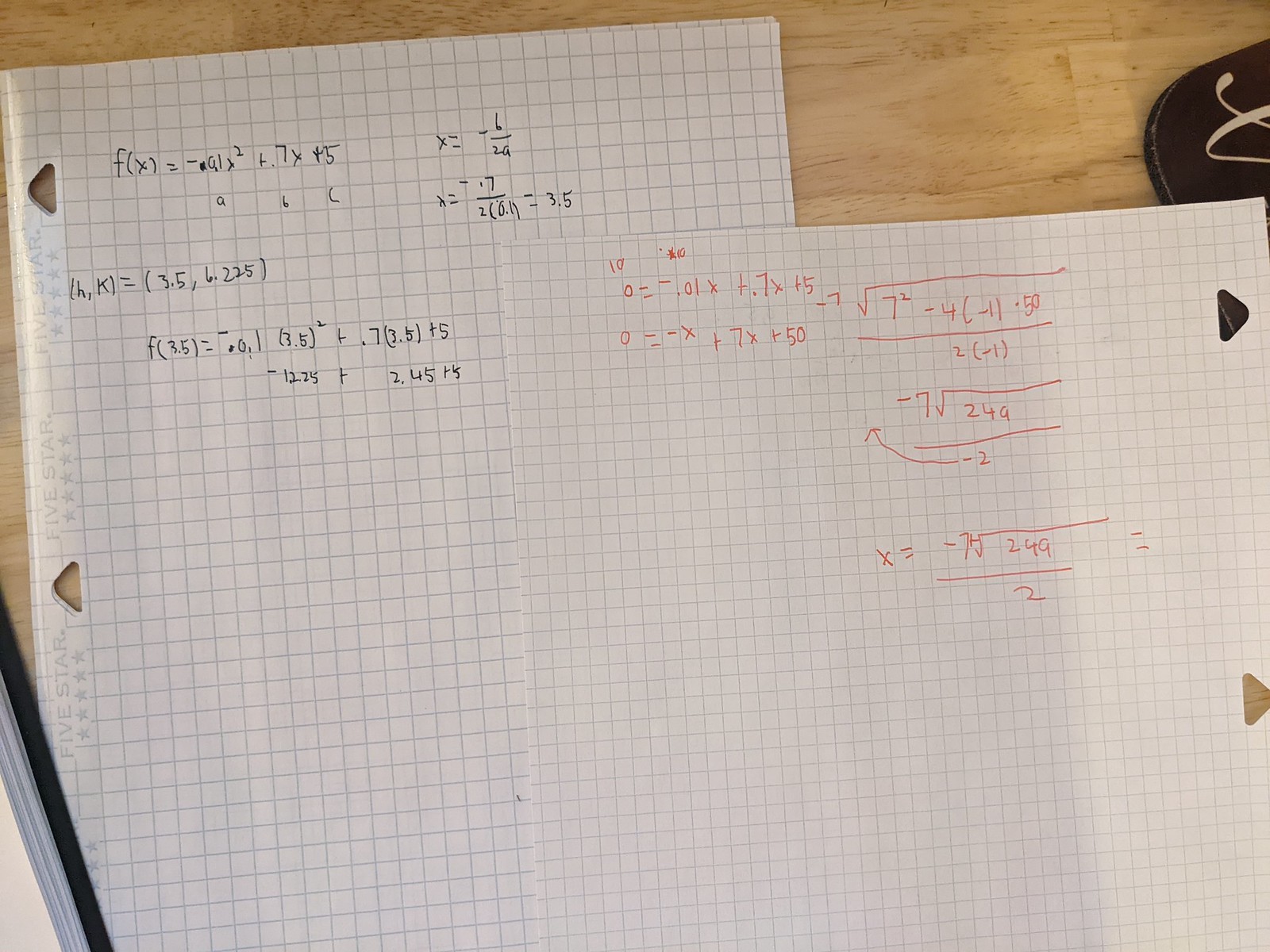On a blonde wooden surface, two pieces of graph paper teeming with complex mathematical equations are arranged such that the top sheet, which bears red ink, partially obscures the bottom sheet, inscribed in black. Both sheets, featuring binder holes on the left side as if torn from a notebook, present intricate and lengthy calculations, evidently striving to solve for X. In the lower left corner of the scene, a glimpse of an open book with a black cover and white pages is visible. Meanwhile, in the upper right corner, a black object with white writing—potentially a mouse pad, wallet, or eyeglass holder—adds an element of intrigue to the meticulous workspace.